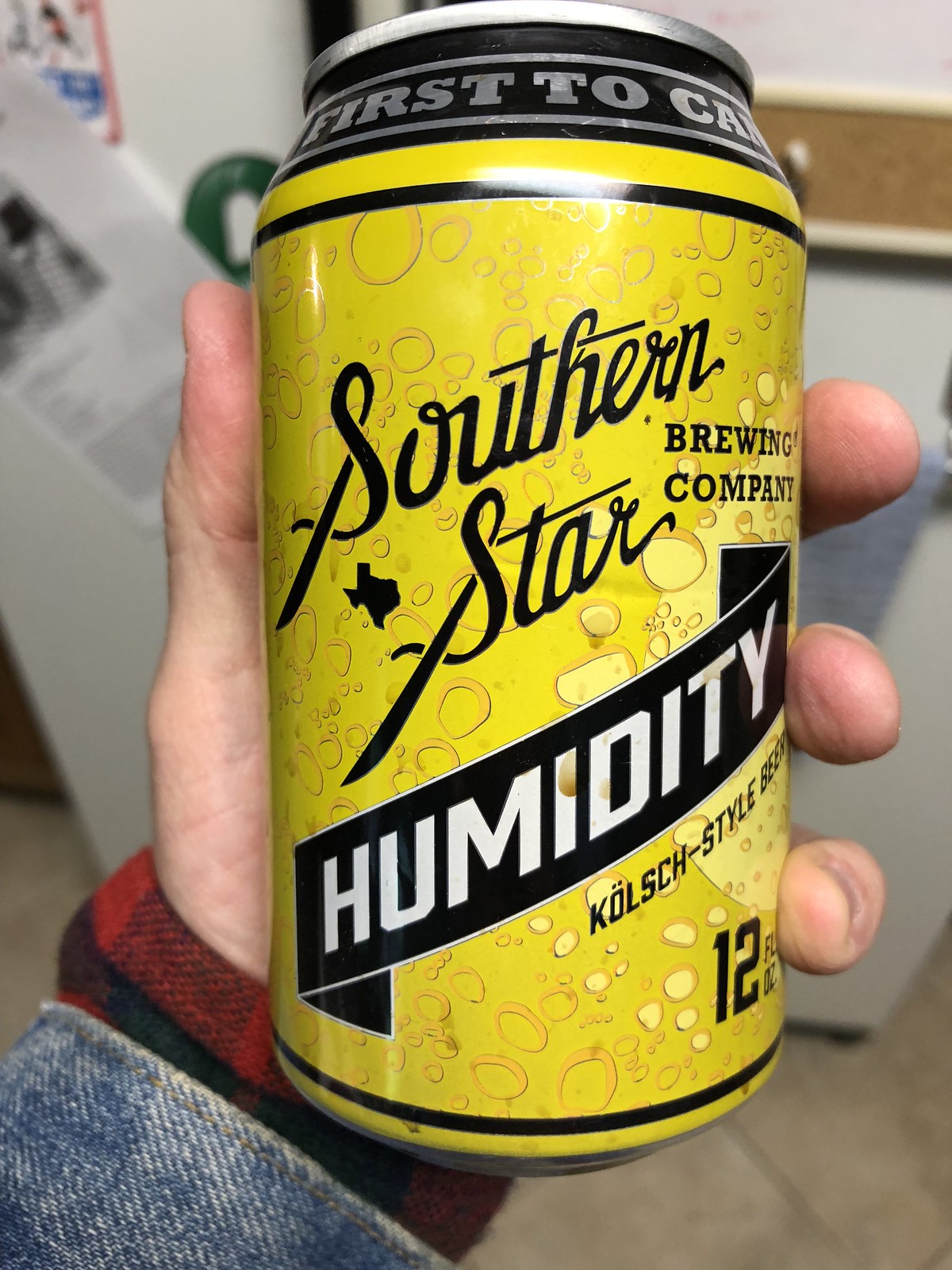In this detailed image, a person is holding a bright yellow can in their hand. The individual is dressed in a red and black plaid long-sleeve shirt with the sleeves extending to cover the wrist, beneath a denim jacket. The background reveals a beige tile floor with visible grout lines, along with white and off-white elements, suggesting pieces of paper or light-colored surfaces. A cork board with lighter wood strips frames part of the scene.

The can itself features intricate design elements: a black top rimmed with silver, transitioning to a yellow body adorned with drawn bubbles. Prominently, it displays the branding "Southern Star Brewing Company" in black letters, with "Southern Star" scripted in a cursive font. Across the midsection of the can is a distinctive black banner bearing the word "Humidity" in bold white letters. Additional text at the bottom of the can indicates "12 fluid ounces" with a black underline. Near the banner, small print in another language is partially visible, adding to the label’s detail.